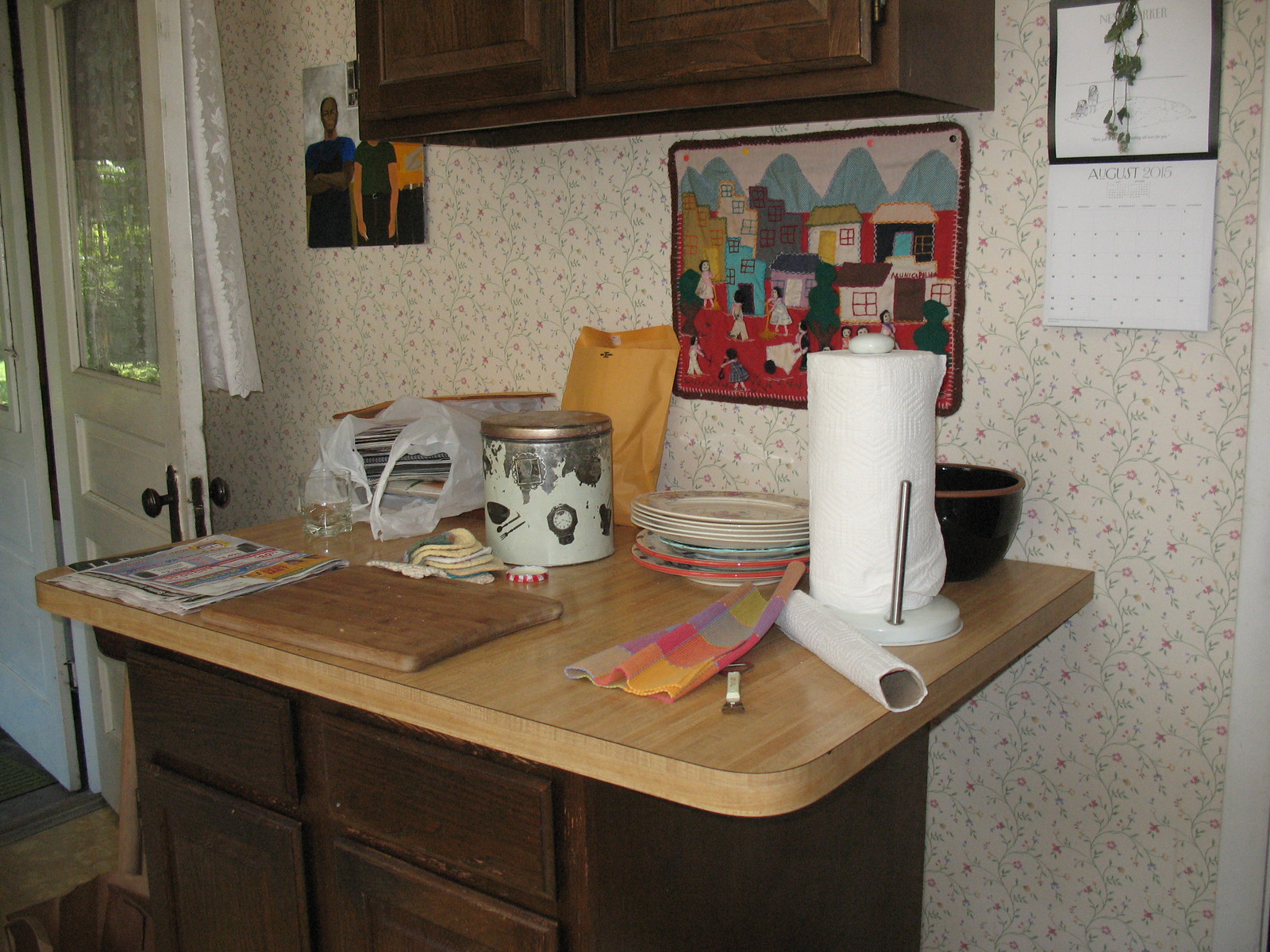This photograph captures a cozy kitchen corner against a tastefully decorated wall. The central feature is a blonde light wooden countertop of a kitchen island set against a vibrant floral wallpaper. The wallpaper combines shades of green, light pink, and white, lending a lively yet elegant ambiance to the space. Below the countertop are darker wooden cabinets that provide a striking contrast. Overhead, additional cabinets of the same darker wood tone add a sense of cohesion to the area.

Hanging above the island is a fabric tapestry displaying houses in various colors—white, blue, gray, and gold. The scene depicted on the tapestry includes children playing in front of the houses, adding a whimsical touch to the decor.

The countertop itself is adorned with an assortment of items. Prominently, there is a white roll of paper towels standing upright alongside an almost empty paper towel roll lying on its side. Behind these rolls, a stack of white plates is visible, accompanied by two plates with a pink rim and a robin's egg blue plate in the middle. A white tin with a bronze-colored lid, featuring what appears to be clock designs, is positioned against the wall. Behind this tin, a manila envelope peeks out. Nearby, a white plastic bag containing some packaging material sits next to a clear glass with a small amount of liquid.

Adjacent to these items is a wooden cutting board, alongside which is a colorful cloth in shades of yellow, pink, orange, gray, and purple. Stacked glossy colored paper lies to one side of the cutting board, while behind it, kitchen cloths in yellow, white, and gray are neatly arranged.

In the background, a white door is visible, adorned with a lace curtain covering its glass window. The wall also features a calendar with a floral image in black and white, enhancing the kitchen's charming and homely feel.